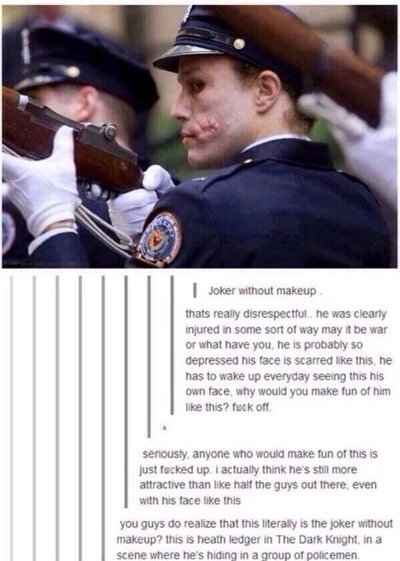The image shows a soldier, likely designed to resemble Heath Ledger's Joker character from "The Dark Knight," posing in a formal, military stance. He wears a blue uniform with a patch on the left sleeve, white gloves, and a military cap. Notably, he has a distinctive scar on his left cheek, reminiscent of the Joker's iconic injury. The soldier is holding a brown rifle, and another similarly dressed soldier stands behind him. In front of him, another figure in white gloves is holding a brown rifle. Below the image, the text reads, "Joker without makeup," followed by an indented series of paragraphs expressing disdain for the caption, highlighting the disrespect implied by mocking the man's injury and emotional state. Vertical lines extend from the left of the text to the bottom of the image, framing the commentary. This appears to be a screenshot from a movie, emphasizing ethical concerns over ridiculing visible trauma.